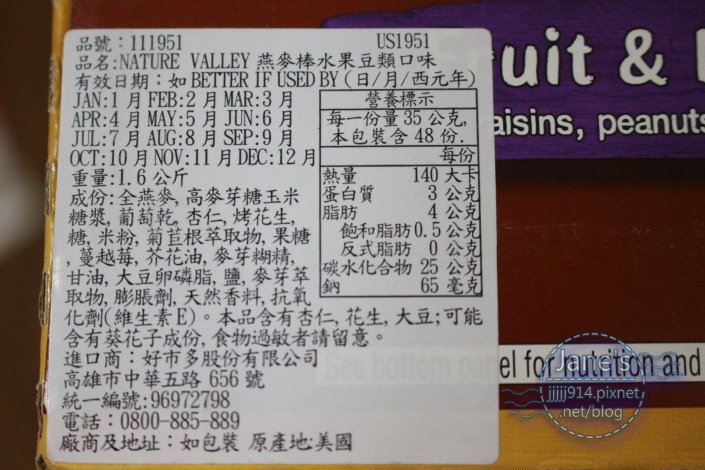The photograph showcases a navy and white box of a product, likely a candy or snack, with a large sticker partially obscuring the box. This sticker contains predominantly Chinese characters, with some English details. The English text includes the brand "Nature Valley" and the phrase "Better if used by" followed by a series of dates: January 1, February 2, March 3, and so forth up to December 12. Visible in white font on a purple section of the label are the words "raisins" and "peanuts." In the background, a partially visible purple sign appears to say "fruit and" or "fruit and nuts." There is also a watermark on the image that reads "James, bunch of J's, 914.pixnet/blog." The white section of the label also features some random numbers and what appears to be some black Asian characters, possibly Japanese.